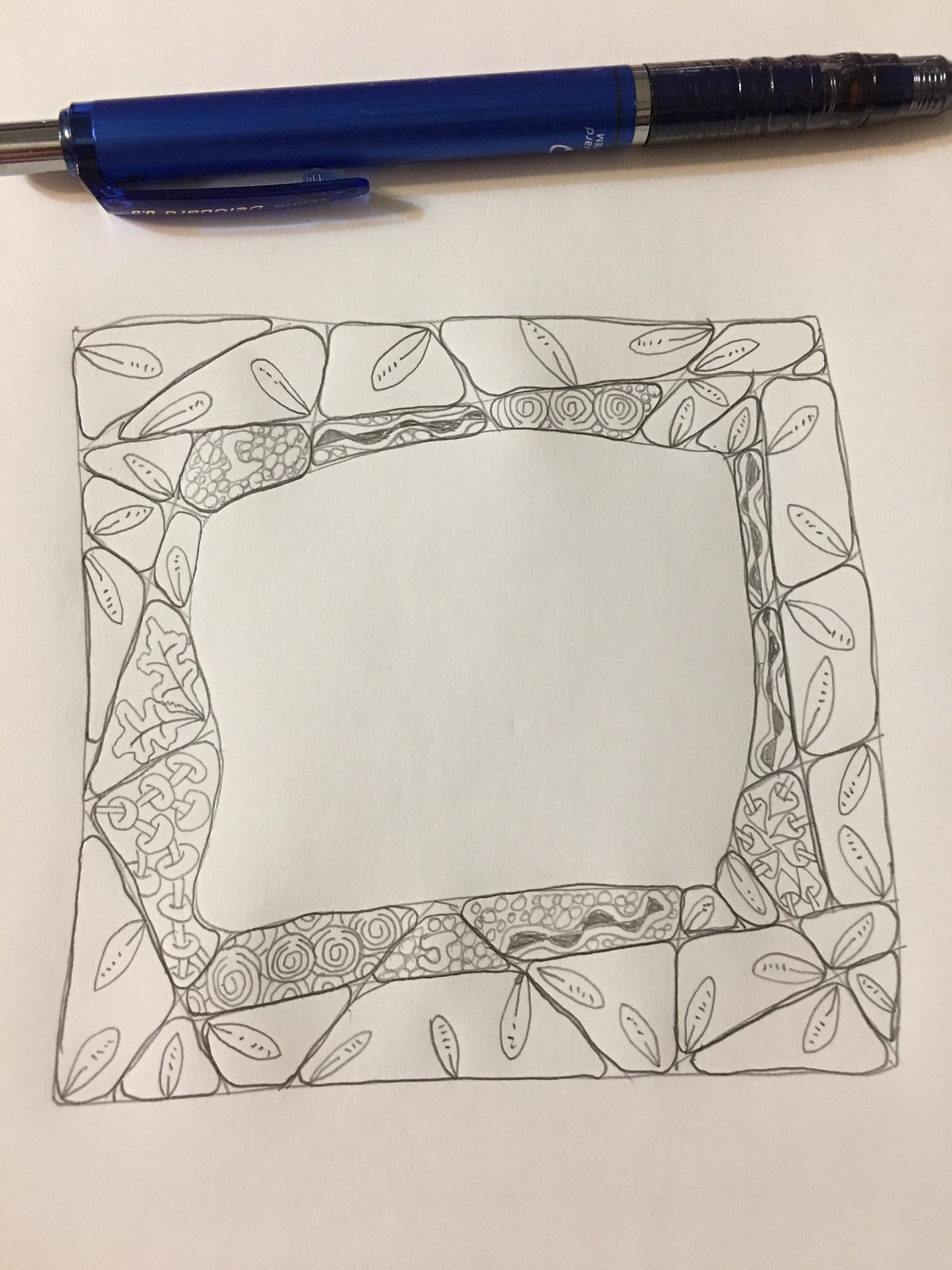The image showcases a color photograph of a meticulously crafted drawing on an off-white vertical sheet of paper. At the top of the photograph is a ballpoint pen, blue on the top and black on the bottom, possibly the tool used to create the intricate design. The drawing itself is square-shaped and ornate, resembling a frame. It features an internal square, creating a layered, geometric pattern. Within this frame are numerous detailed illustrations of leaves, distributed across what appear to be triangular segments pieced together to form the larger square motif. The overall design gives the impression of a finely detailed, nature-inspired frame, executed with precision, possibly in pen or pencil.